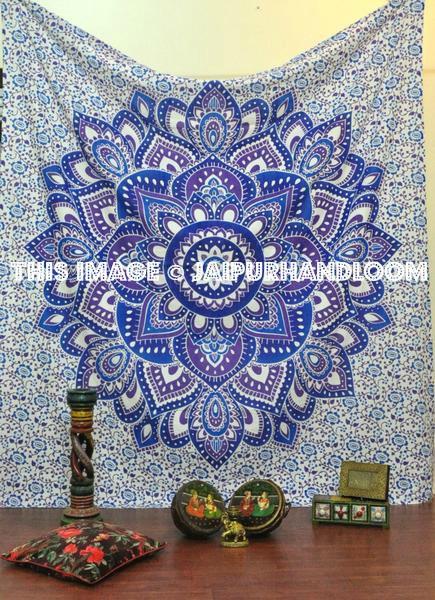This image showcases a vibrant Indian tapestry or blanket, predominantly adorned with shades of blue, purple, and white. The tapestry features a large, intricate mandala design that dominates approximately 70% of its surface, with a central blue circle surrounded by layers of blue and purple petal-like shapes, progressively expanding outward. Encircling the mandala are ornate patterns of delicate blue flowers and purple leaves connected by elegant vines.

Hanging on the wall, the tapestry serves as the backdrop for a mid-dark stained furniture top at the bottom of the image. The tabletop is adorned with several items such as a square velvet floral pillow, a green, yellow, and red candlestick devoid of a candle, a small brass elephant figurine, and a decorative jewelry box topped with a gold picture frame.

Additionally, the tapestry features the text "Jaipur Handloom" with a copyright symbol situated at its center. On either side of this central text, there are vintage-looking pictures—one on the left showing a couple dressed in orange and green, and another on the right depicting a couple in red and green. Below these images lies a statue of an animal and an item with four squares, contributing to the rich, cultural ambiance of the scene.